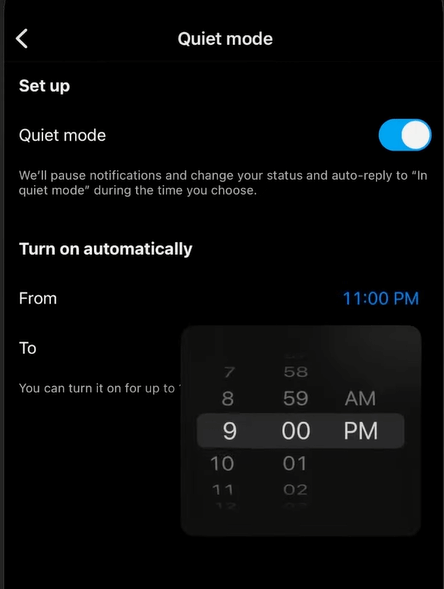A detailed screenshot of a mobile phone displaying the setup for Quiet Mode in Dark Mode. At the very top, the text "Quiet Mode" is prominently featured. To the side, the word "Setup" is in bold, indicating a configuration process. Below, the term "Quiet Mode" is repeated alongside a switch button, which is currently toggled to the "on" position.

The description beneath the switch reads: "We'll pause notifications and change your status to 'In Quiet Mode' and auto-reply during the time you choose." There's an option to "Turn on automatically from 11 p.m. to..." with the dropdown time menu currently adjusted to select 9 p.m., illustrating that this user is setting their Quiet Mode to last for 22 hours. Some text specifying additional details is partially obscured by the selection, showing: "you can turn it on for up to..." with the latter part cut off.

The page uses Dark Mode, with a black background and white text, providing a visually comfortable display especially in low-light conditions. Notably absent are typical status indicators like the current time, signal strength, or battery life, focusing solely on the Quiet Mode setup screen. The user is essentially configuring their phone to remain in a silent, undisturbed state for the vast majority of each day.